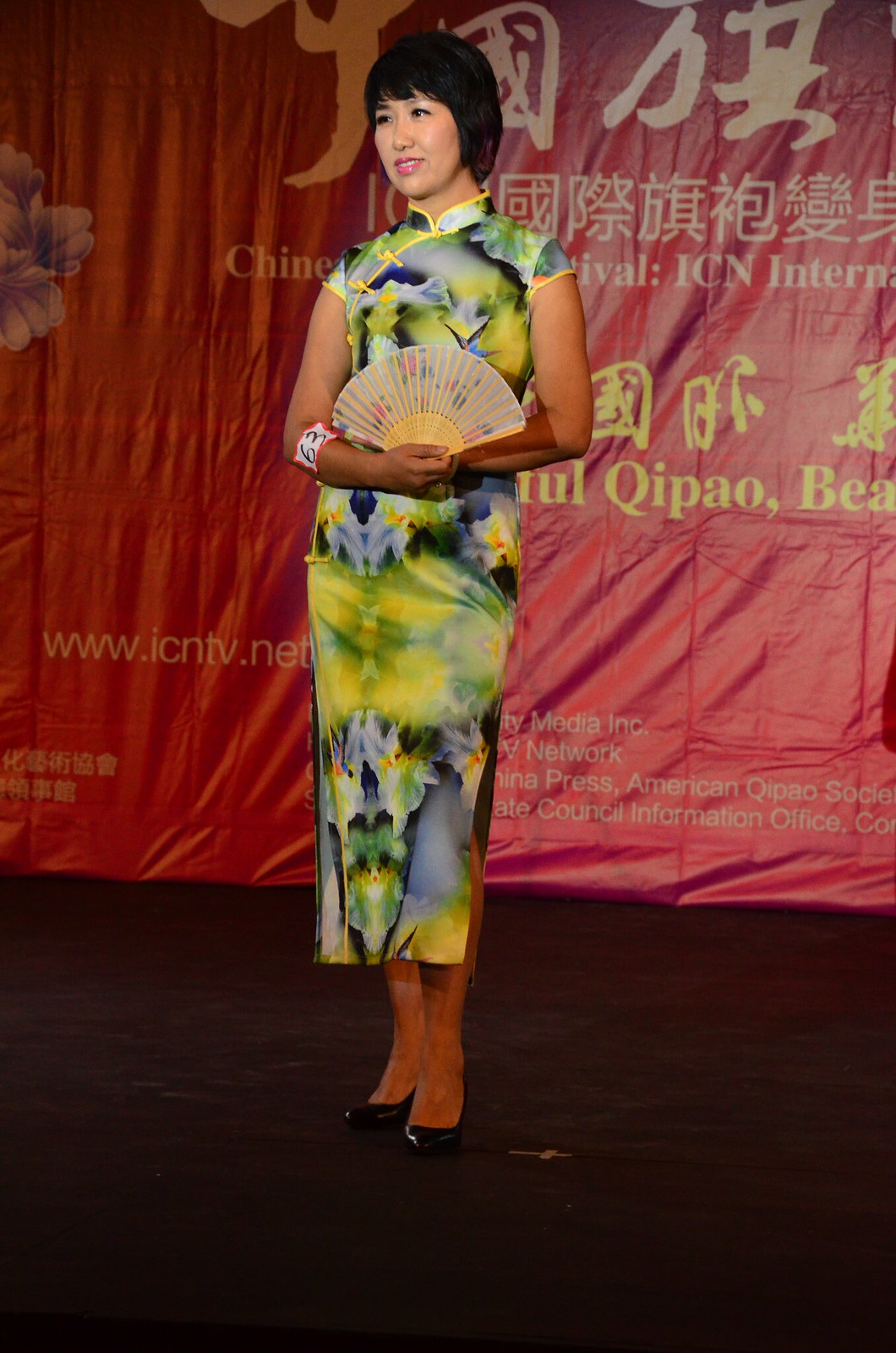In this image, an Asian woman is standing on a stage in front of a vibrant red backdrop adorned with numerous Chinese characters and the website address www.icntv.net in yellow. The backdrop also reads "Chinese Festival ICN International" and features a flower design in a darker red hue to the left. The woman has chin-length black hair with bangs and wears a short-sleeved, calf-length dress with a mandarin collar. The dress is a blend of green, yellow, light blue, and black, resembling a tie-dye or watercolor floral pattern. She holds an open paper fan with both hands, positioned in front of her waist. A white rectangular band with the number "63" printed in black is worn high on her left forearm near the elbow. She pairs the dress with black high heels and has a slight smile on her face, exuding a poised and elegant demeanor.